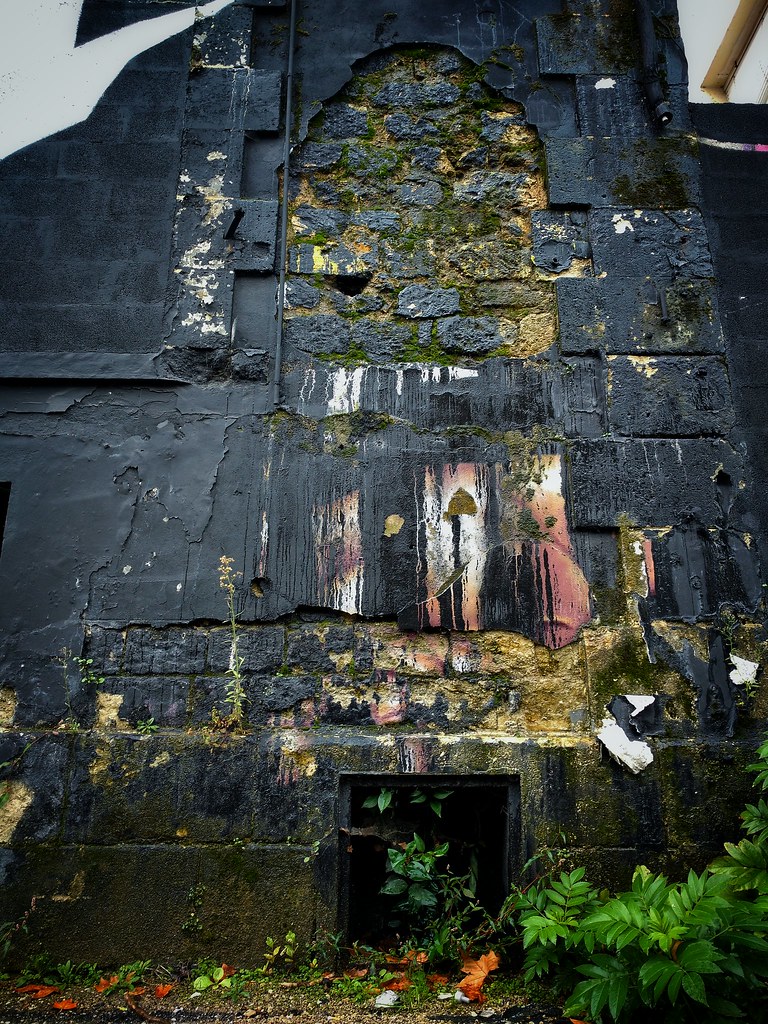This is a vertically aligned photograph of a very old, abandoned stone building. The structure has an aged appearance with visible signs of wear and deterioration. The building is made of large black stones, some with chunks of the facade peeling or chipped off, revealing dark gray stones beneath. The surface is streaked with pink and green, likely from moss or mildew that has taken hold over the years. The upper left corner of the image shows a sliver of a gray, cloudy sky. 

In the middle of the building, moss and foliage have spread extensively, creating a rich patchwork of greenery against the dark stone. Toward the bottom, you can see the base made of large, horizontal rectangular stones. There is a tall, squarish opening at the base, appearing as a dark, inviting entrance into the dilapidated structure. The interior looks pitch black, giving a sense of depth to the abandoned space.

At the bottom of the image, the ground is a mix of dirt, scattered orange and green leaves, and various plants. The lower right corner features a dense area of green branches and leaves, adding to the scene's overgrown, untended atmosphere. The overall impression is one of a once-sturdy edifice now overtaken by nature, standing in quiet testament to the passage of time.